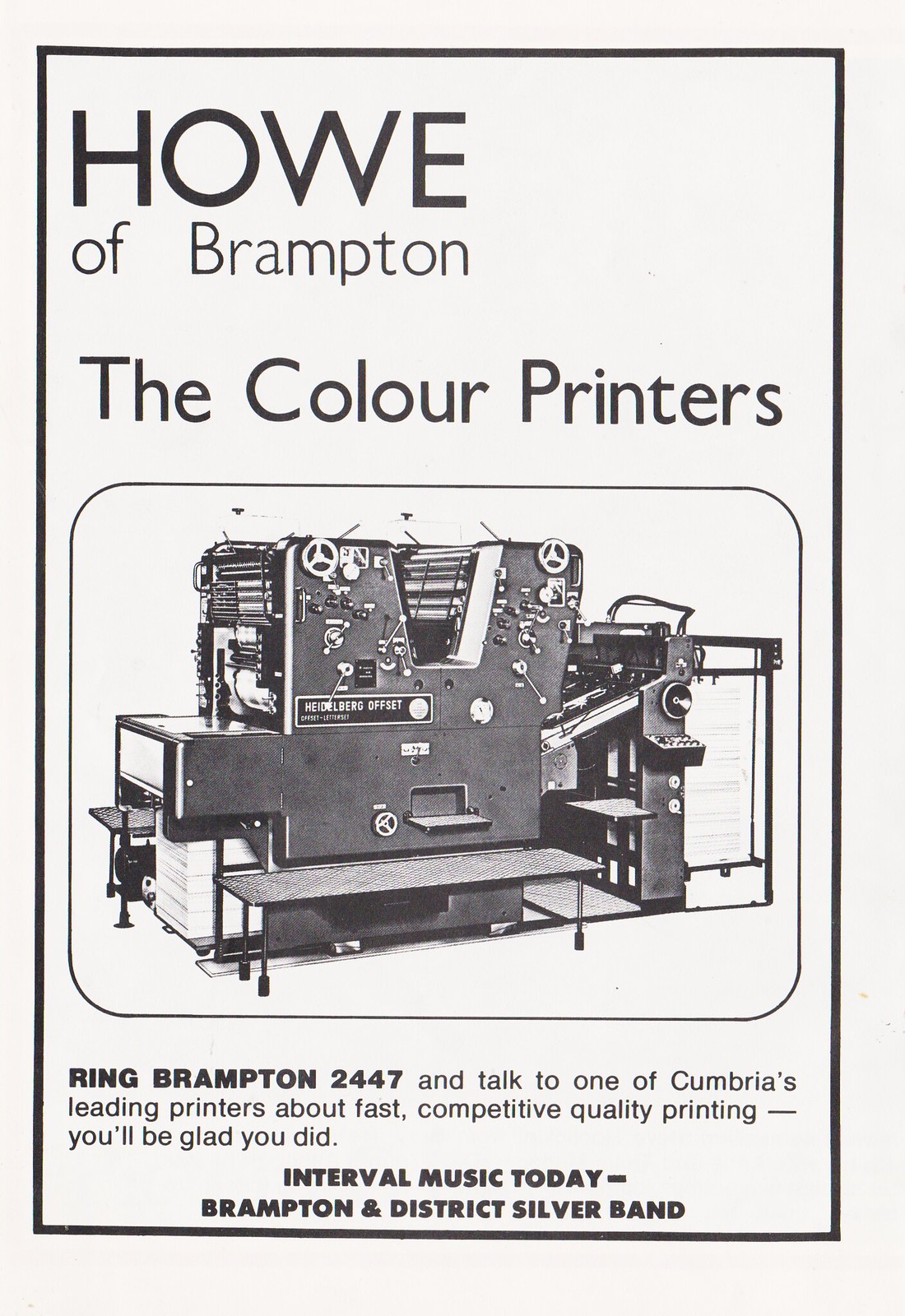The image is an older advertisement, possibly from a magazine or a poster, for Howe of Brampton, The Color Printers. The advertisement is presented on off-white paper with a black border and features predominantly black lettering. At the top in large black letters, it reads "Howe of Brampton" with "The Color Printers" directly underneath, despite the entire advertisement being in black and white. Below this text, there is a large black and white photo of a professional-grade printing press, likely used for newspapers or similar large-scale printing tasks. Under the image, bold text reads, "Ring Brampton 2447 and talk to one of Cumbria's leading printers about fast, competitive, quality printing. You'll be glad you did." At the very bottom of the advertisement, also in bold, uppercase letters, is the text, "Interval Music Today, Brampton and District Silver Band."